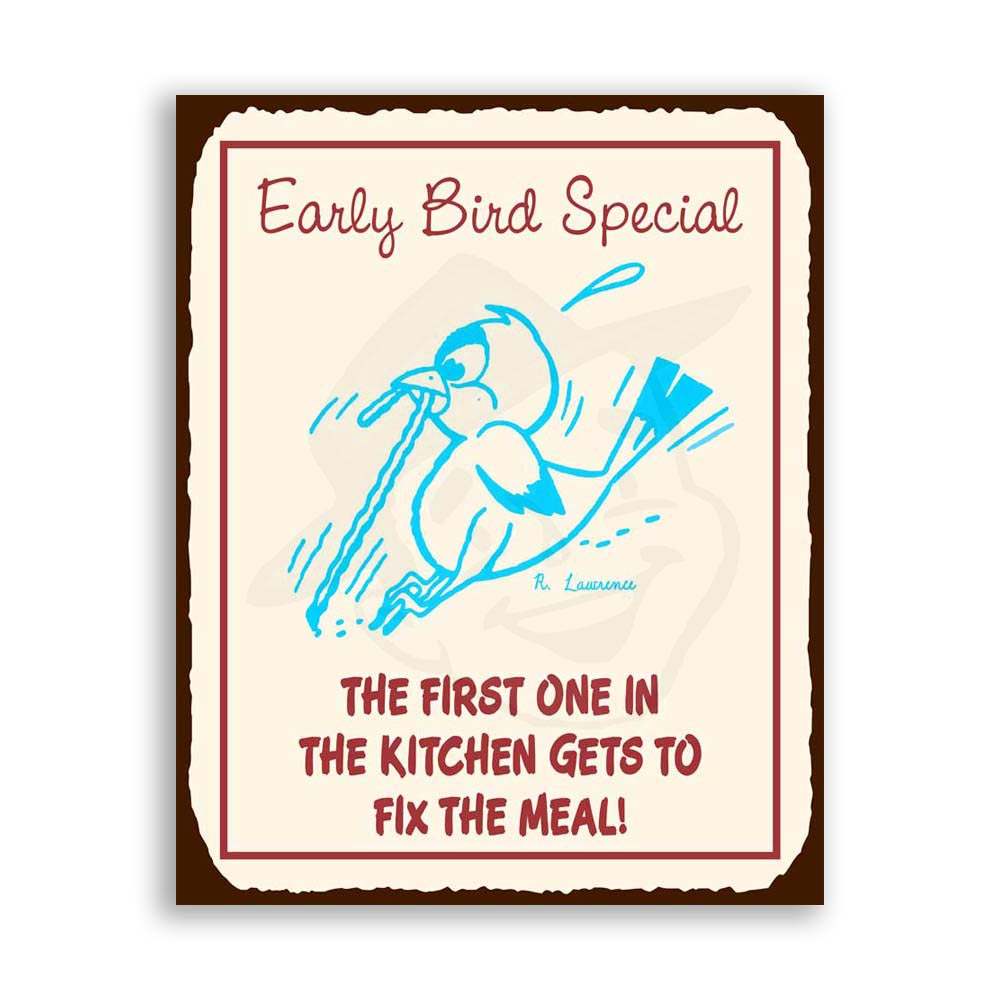This image features a framed restaurant advertisement on a white page with a detailed design. The outer border of the advertisement is deep brown, transitioning into a beige interior. At the top, bold red letters announce "Early Bird Special," accompanied by an animated baby blue outline of a bird. The bird, shown straining with sweat drops and effort lines, attempts to pull a worm from the ground. Below this central image, the text humorously states, "The first one in the kitchen gets to fix the meal!" Adding to the whimsical nature of the sign, a faded watermark in the background depicts a young boy wearing a brimmed hat, smiling. The artist, R. Lawrence, has signed the artwork. Overall, the playful illustration and clever text convey a lighthearted message, likely intended to entice diners with the promise of a special deal for early arrivals.